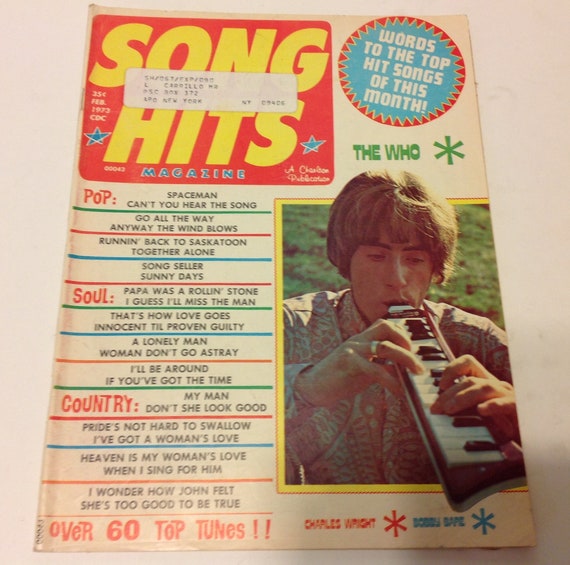The cover of this vintage magazine features a prominently placed white post office label with an address at the center. In the top left corner, "Song Hits" is displayed in bold yellow letters against a red background, with "Magazine" written underneath. A blue circular bubble with a sawtooth border in the top right corner reads "Words to the Top Hit Songs of the Month". Below this, in green letters with a small star, is "The Who," and beneath it, an image of The Who's lead singer playing a small keyboard-like wind instrument while wearing a floral long-sleeve shirt. To the left of this image, a vertical list details various top songs, categorized into pop, soul, and country genres. At the bottom of the cover, "Over 60 Top Tunes" is printed in red, next to the name "Charles Wright" and a partially legible name, possibly "Bobby something," accompanied by small stars.